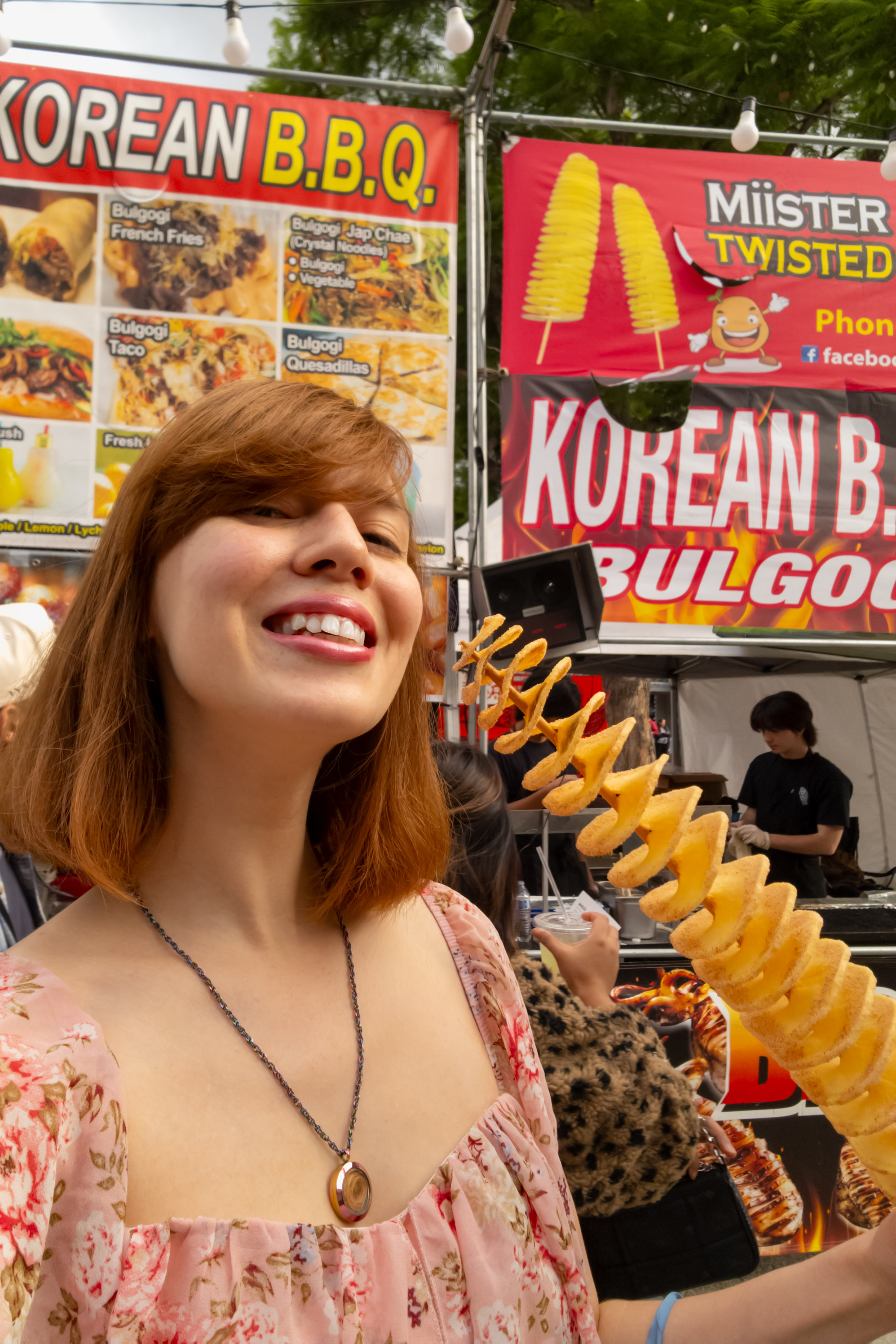A vibrant photograph captures a moment at what seems to be a bustling street fair or food festival. The central figure is a woman with straight ginger hair, adorned with red lipstick, smiling warmly at the camera. She is dressed in a pink, floral-patterned dress and wears a delicate necklace with a pendant. In one hand, she proudly holds a food item, a spiral-shaped, yellow fried potato skewer from a vendor called "Mr. Twisted."

Behind her, vivid banners advertise street food delicacies. One notable banner in white font on a red background reads “Korean BBQ,” accompanied by enticing images of various dishes including Korean Bulgogi. Another banner also announces "Mr. Twisted." Further back, street shops teem with activity, and a tree subtly frames the vibrant scene, adding a touch of greenery to the lively outdoor setting.